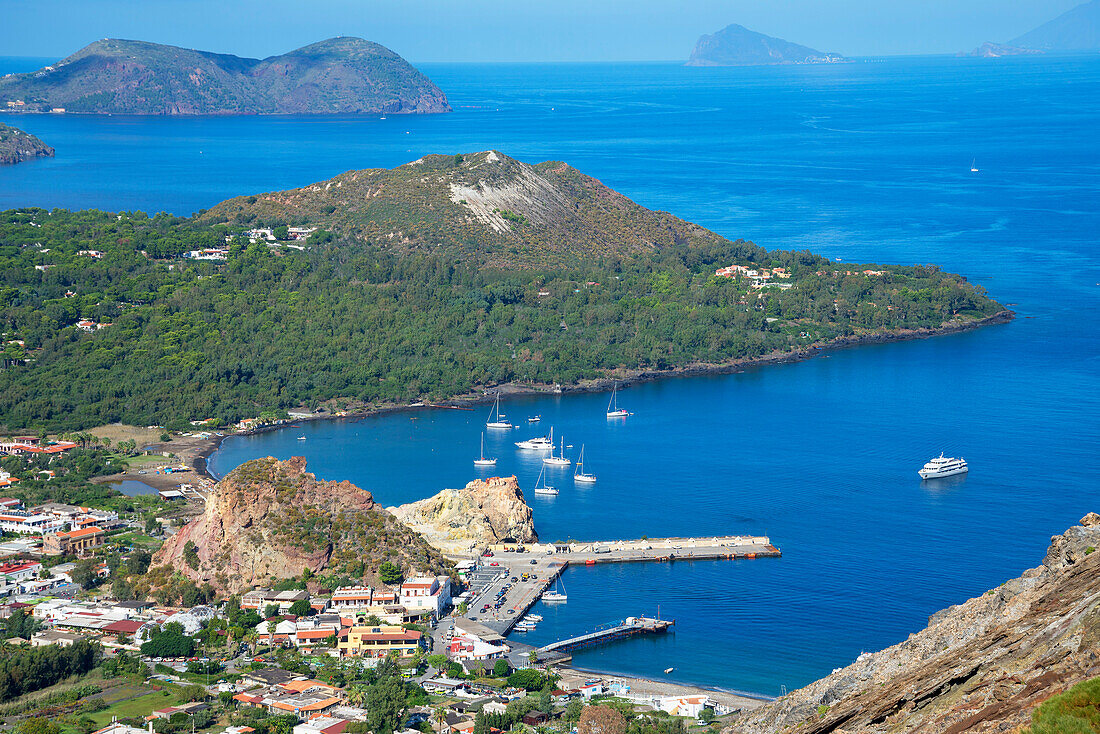This outdoor aerial photograph, likely taken from a drone or airplane, vividly captures a large, tropical seaport set against a backdrop of a mesmerizing ocean in varying shades of blue. On the left side of the image, a peninsula extends out into the bright blue water, almost reaching the right edge of the photograph but leaving a channel of water in between. The peninsula is densely covered in lush trees of various green hues and features a distinctive beige patch running down a hillside or small mountain.

At the center-left portion of the photograph lies a bustling seaport with a long, wide dock extending horizontally towards the right. This marina area hosts multiple white sailboats and a small to medium-sized cruise ship that appears to be either departing or arriving. Behind the seaport, in the lower left corner, there is a quaint town or village with various small buildings and a road leading up to the coast.

Surrounding the seaport and extending out towards the upper center of the image is a vegetated, hilly area that forms a natural harbor. In the background, a striking blue ocean stretches out, punctuated by distant, misty islands and a small atoll towards the upper right. The horizon line is close to the top of the photograph, capped by a bright blue sky that seamlessly complements the water below. Additionally, another tall, lush hillside rises up from the sea in the upper left corner, adding depth and a sense of tropical serenity to the scene.